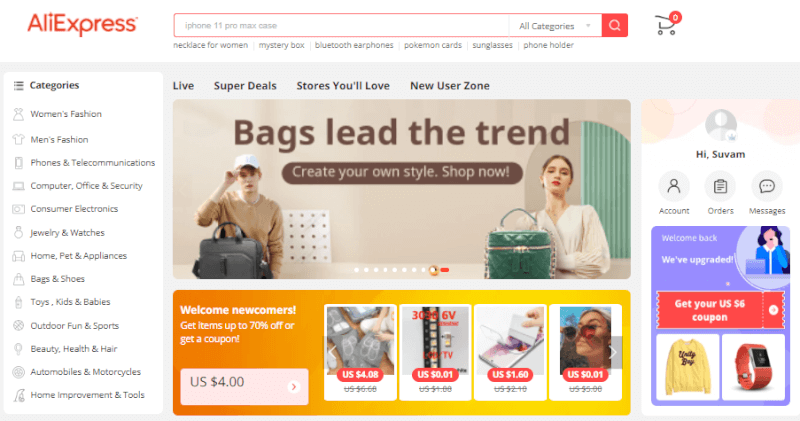This screenshot captures the homepage of the AliExpress website in detail. The AliExpress logo, displayed in distinctive orange, occupies the top left corner of the screen. Adjacent to it on the right, there is a comprehensive search bar that facilitates category selection and highlights trending search terms. Moving further right, you can see an icon representing a shopping cart, accompanied by a numeral indicating the count of items in the cart. 

On the left-hand side of the interface, a vertical category banner is visible, listing an extensive array of categories such as Women's Fashion, Men's Fashion, Phones & Telecommunications, Computer, Office & Security, Consumer Electronics, Jewelry & Watches, Home, Pet & Appliances, Bags & Shoes, Toys, Kids & Babies, Outdoor Fun & Sports, Beauty, Health & Hair, Automobiles & Motorcycles, and Home Improvement & Tools.

Centrally positioned on the page are additional categories like Live, Super Deals, Stores You'll Love, and New User Zone. The most prominent element in this section is the main banner, adorned with stock images of models holding handbags. The banner promotes the message: "Bags lead the trend, create your own style shop."

Supplementary promotional banners are situated at the bottom and on the right side of the screen, displaying various items on sale. The top right corner of the homepage hosts the user interface features, including icons for Account, Orders, Messages, and an image of the user's profile.